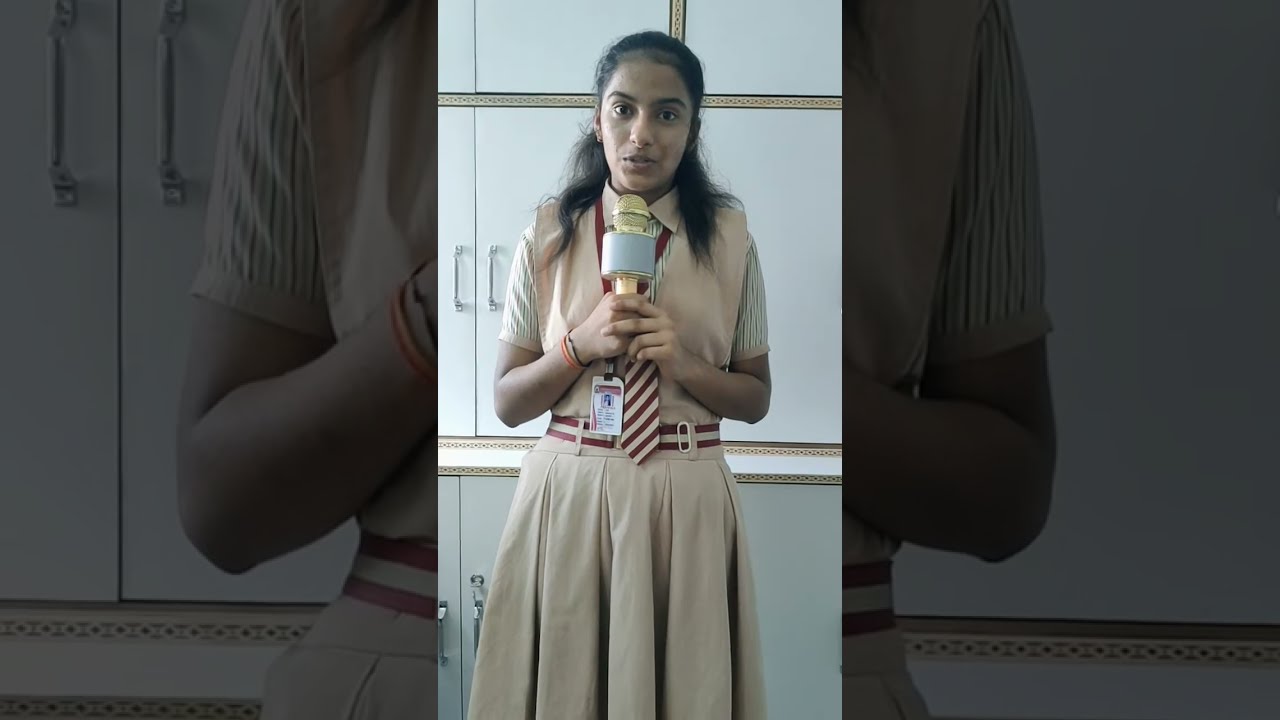This horizontal rectangular image prominently features a young woman, likely a student, speaking into a gold-colored microphone. Positioned centrally, the woman stands out with a vertical, rectangular section in color. She is wearing a light tan dress with a pleated bottom and a matching tan vest with red accents on the V-neck. A red and tan belt, with a brass buckle, cinches her waist, and her brown and red striped tie enhances the academic uniform appearance. She has longer black hair that spills over her shoulders, smooth yet wispy, and slightly darker skin, perhaps hinting at Hispanic, Middle Eastern, or Indian descent. Her mouth is open, revealing her teeth, as she speaks confidently into the microphone.

On her chest, she wears something that suggests an identity card holder, enhancing her scholarly demeanor. The left and right sides of the image contain close-up, zoomed-in views of her body, each shaded in black, adding a sense of depth and focus on the central portrait. Behind her is a background of white cabinets with gold trim, contrasting with the darker, almost faded surroundings that frame her.